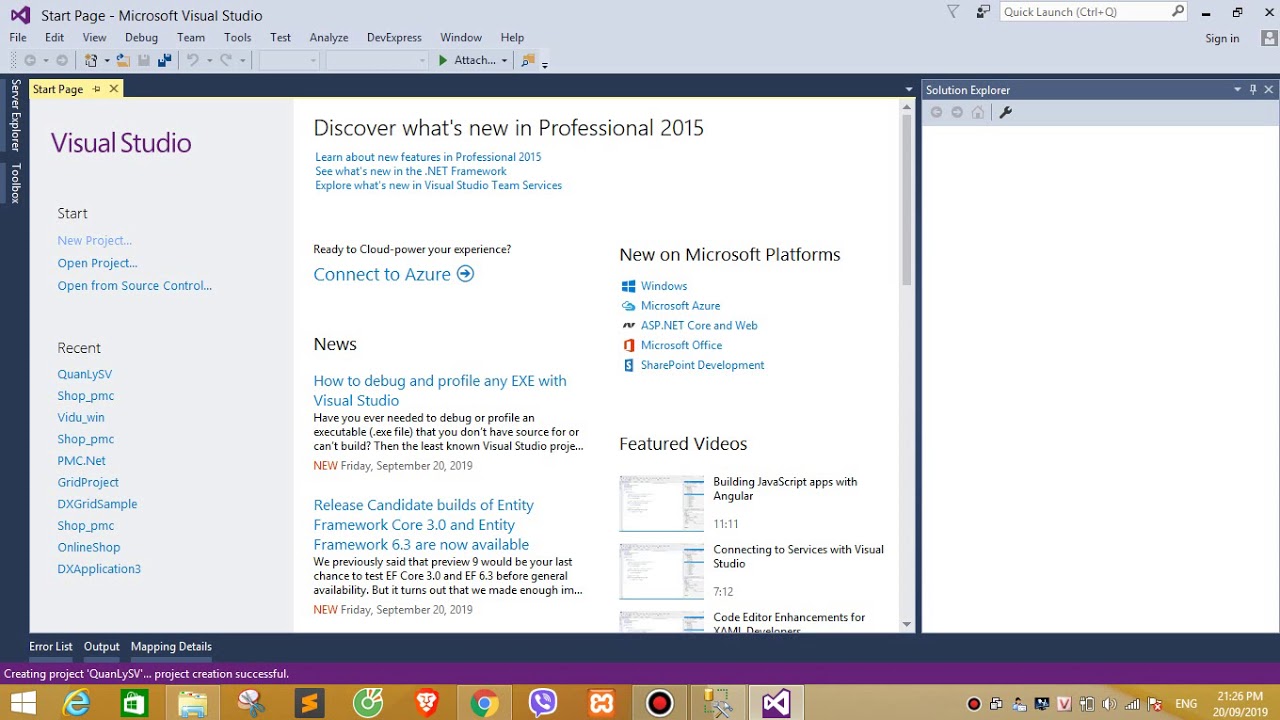This is a detailed description of a web page for StarPage in Microsoft Visual Studio. At the top border, there is a Quick Launch box next to a drop-down symbol, a maximize screen button, and a close button.

On the top-right corner, there's a "Visual Ed" sign-in area featuring a placeholder for a user photograph. The menu bar includes tabs for File, Edit, View, Debug, Team, Tools, Test, Analyze, DevExpress, Window, and Help. Below the menu bar, there are icons for duplicating, saving to disk, opening a folder, and navigating left or right through code changes.

In the main content area, "StarPage" is prominently displayed with a "close-out" X next to it and "Visual Studio" in blue text on a gray background. It provides quick actions such as "Start New Project," "Open Project," and "Open from Source Control." Recent projects listed include QuantiSV, shop.pmc, vidu.win, shop.pmc, pmc.net, GR, Grid Project, DX Grid Sample, shop.pmc, shop_PMC Online Shop, and DX Application.

To the right of these options, it says "Discover What's New in Professional 2015" with subtitles that are hard to read. Below this, the section titled "Ready to Cloud Power Your Experience" elaborates on the latest Microsoft platforms, including Windows, Microsoft Azure, ASP.NET Core and Web, Microsoft Office, and SharePoint Development.

At the bottom left of this section is "News," highlighting an article titled "How to Debug and Profile Any EXE with Visual Studio." Beneath that, updates about the "Release Candidate Builds of Entity Framework Core 3.0 and Entity Framework 6.3" are mentioned.

Additionally, there are feature videos on "Building JavaScript Apps with Angular," "Connecting to Service with Visual Studio," and "Code Editor Enhancements." At the very bottom, there are typical desktop icons including Microsoft Edge, Windows Explorer, a folder, Clipboard, Google Chrome, and a phone, among others.